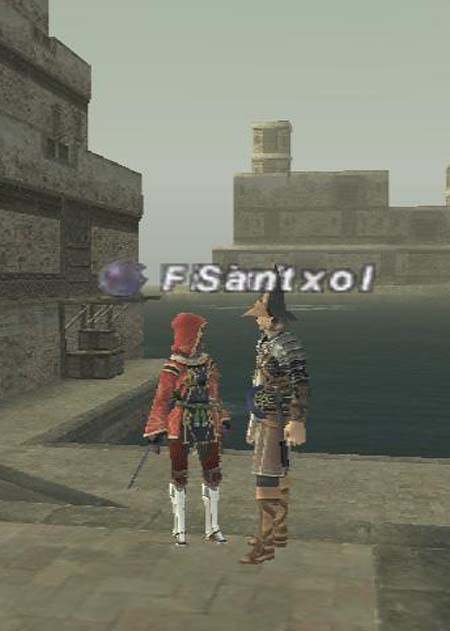This is a detailed screenshot from the video game Final Fantasy XI Online. The overall color palette of the image consists mainly of varying shades of brown. On the left side, there's a tan building accented with darker brown tones. The ground is composed of stone tiles in a light tan hue, indicative of a port setting. In the background, you can see blue water and another tan building positioned at a distance, under a cloudy gray sky.

In the foreground, there are two characters standing close to each other. The character on the left is adorned in samurai-style armor on the upper half, complemented by a witch's hat and tan boots. The character on the right is dressed in red robes with a matching hood, paired with white boots. Above their heads, white lettering spells out "F-S-A-N-T-X-O-L".